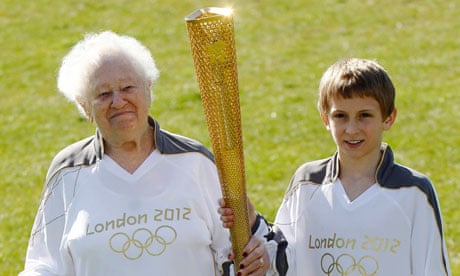The image shows an older woman and a young boy standing on a bright green grassy field, both visible from the waist up. On the left, the woman, with short, curly white hair, wears a white top adorned with blue fabric at the shoulders and gold lettering that reads "London 2012," along with the gold Olympic ring logo beneath. She is gripping the Olympic torch with one hand. Beside her on the right is a young boy with short brown hair, dressed in an identical top. He holds the same golden Olympic torch slightly higher up, making it positioned centrally between them. Both individuals appear to be celebrating or participating in an Olympic event, symbolizing unity and continuity between generations.